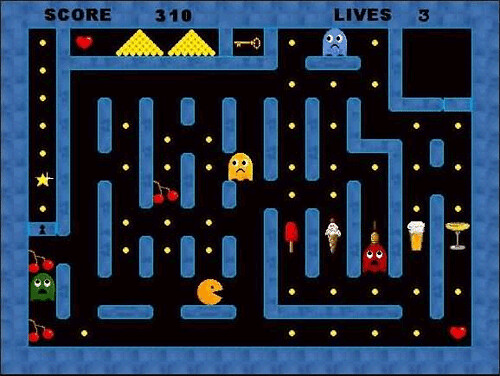A classic Pac-Man game screen is depicted against a black background with blue borders and maze walls. At the center of the maze, Pac-Man, the iconic yellow character, navigates through the pathways. Cherries, ice cream cones, milkshakes, martinis, and popsicles are scattered throughout the maze, serving as collectible items that Pac-Man must consume to earn points. The maze is also inhabited by colorful ghosts, the antagonists of the game, who pursue Pac-Man in an attempt to thwart his progress. Notably, the simplicity of Pac-Man's design contrasts with the more complex figures of the various items and ghosts, emphasizing him as the hero of this enduring arcade classic.